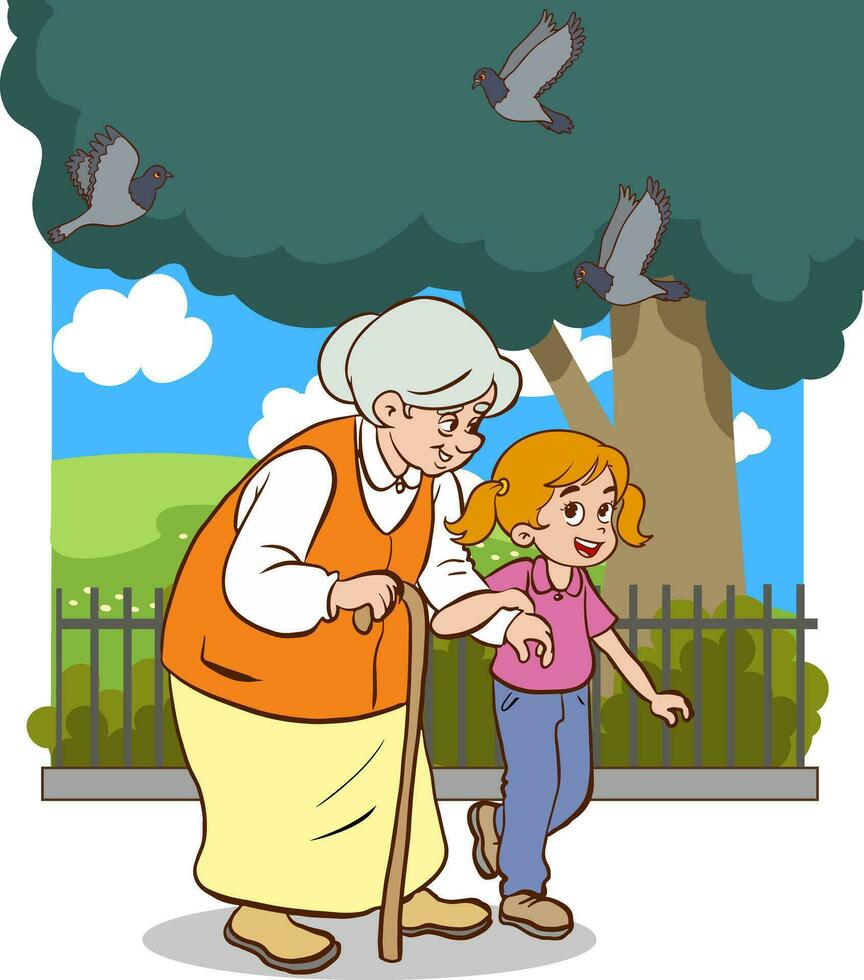The image is a charming cartoon-style depiction of an older woman and a young girl, likely grandmother and granddaughter, walking together along a park-like setting. The backdrop features a lush green hill, a bright blue sky adorned with puffy cotton ball clouds, and a large tree with a dark green canopy. Three pigeons are seen flying overhead, adding to the tranquil city park atmosphere. Separating the greenery in the park from the foreground is a wrought iron fence. The grandmother, who sports gray hair, is dressed in a yellow skirt, an orange vest, and a white blouse. She is holding a cane as she walks. The young girl, with her orange hair styled in pigtails, is wearing blue jeans and a pink blouse. She holds onto her grandmother’s arm tenderly as they stroll.